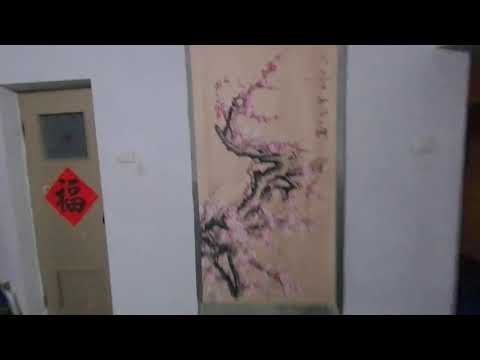The image, seemingly taken indoors at a school in Japan, displays a white-walled room with specific architectural and decorative details. On the left side, there is a cream-colored steel door featuring a small covered window at the top and a vent at the bottom. The door is adorned with a distinctive red diamond-shaped sign displaying black Japanese characters. Centrally prominent on the otherwise white wall is a rectangular banner or wall hanging. This banner showcases a detailed illustration of a branch with cherry blossoms, boasting pink petals against a cream background and a gray border. The blossoms appear intricately drawn along twisty, greyish branches. The photo, albeit dark and of low resolution, captures these elements with considerable detail, representing a typical Japanese indoor scene.